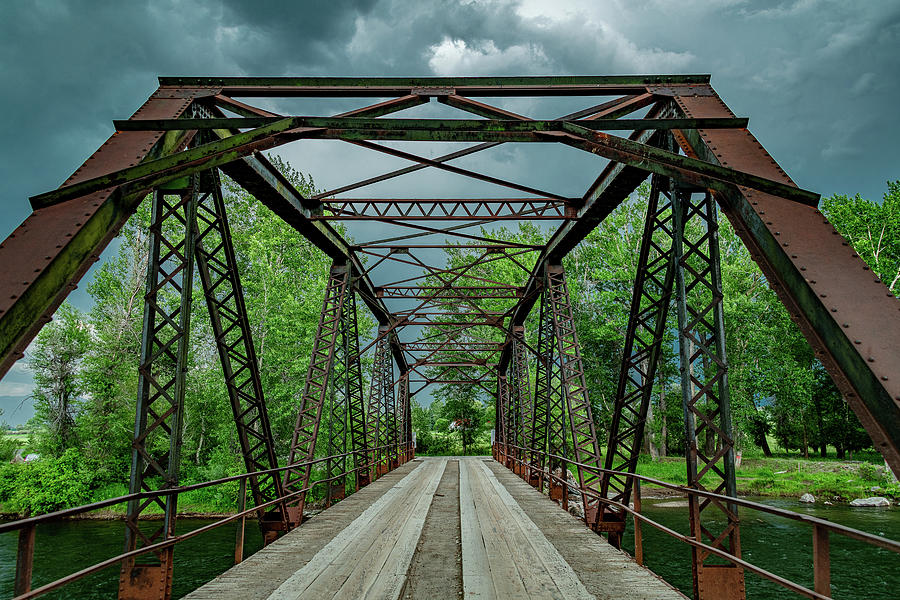This photograph features an old, weathered bridge with a distinctly rust-colored, dark brown hue. The bridge is designed with intricate lattices and triangular trusses that contribute to its sturdy, albeit aged, appearance. Covered in wood planks of varying shades, from dark to light, the bridge narrows enough to suggest it's meant for pedestrian use rather than vehicular traffic. It stretches over a dark blackish-blue body of water, possibly a small lake or pond, and leads to a lush landscape of vibrant green trees and fields. The sky above is completely overcast with a dark gray tone, lightening slightly at the center, giving a sense of impending rain or a storm. The bridge's lower sections, especially near the water, exhibit significant rust. The scene evokes a strong mood of gloominess and nostalgia, reminiscent of a setting from the movie "Stand By Me," with visible rivets and metal trusses adding to the industrial, old-world charm.